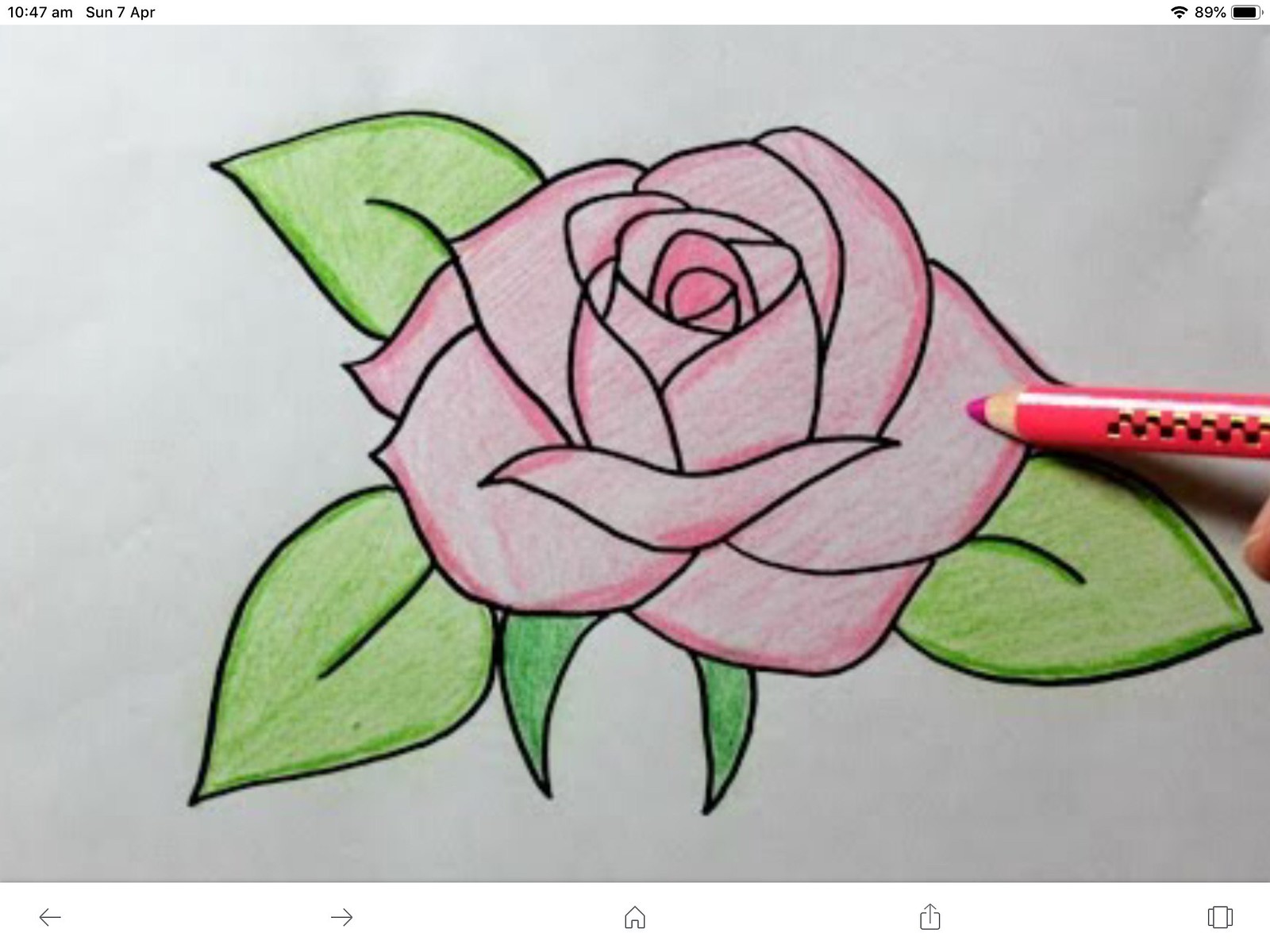The image depicts a detailed, color drawing of a fully bloomed pink rose with meticulously outlined petals and leaves, created with colored pencils. The rose exhibits a gradient of light pink and white shades, with its center fully colored in pink. Surrounding the rose are five distinct leaves—three larger green leaves positioned on the right, upper left, and bottom left of the rose, and two smaller ones near the nonexistent stem. On the right side of the image, there's a pink colored pencil, featuring a gold checkered design, being held by a person, with the tip of their finger and a hint of their white fingernail visible.

The drawing is on a white piece of paper, and the photograph itself is a screenshot from a mobile device. In the upper right corner of the screenshot, a Wi-Fi symbol, an 89% battery icon, and the battery percentage are visible. The upper left corner displays the time as 10:47 AM and the date as Sunday, April 7. The bottom of the screenshot shows typical phone navigation icons including left and right arrows, a home button, a share button, and potentially a call button.